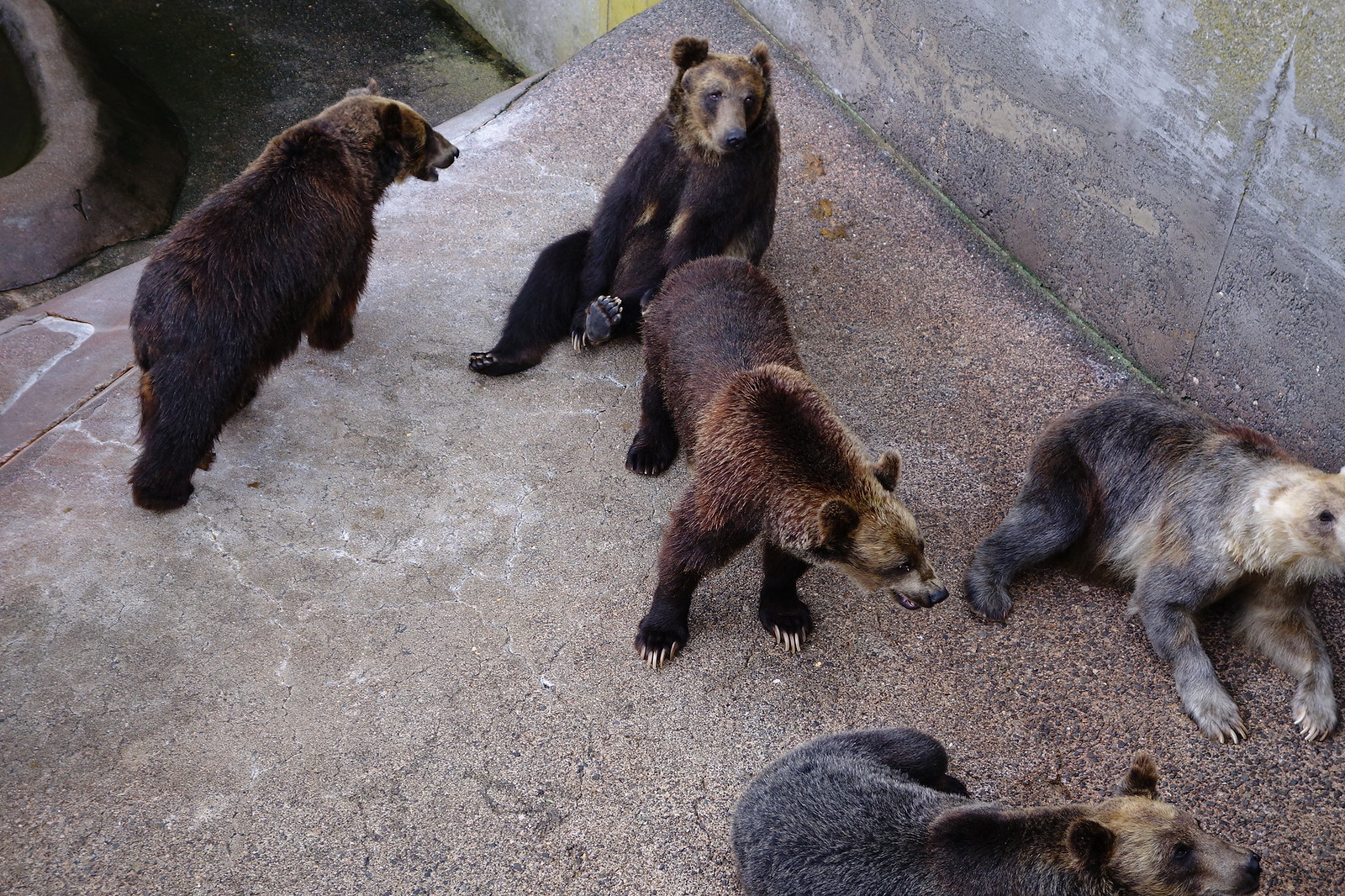The photograph captures a group of five grizzly bears within a zoo or wildlife reserve enclosure. The bears are primarily dark brown with varied fur colorations, exhibiting light brown and gray patches. All five bears are stationed in a small, concrete sunken pit, creating a somewhat confined atmosphere. The enclosure is visible with plain concrete walls and possibly a lower sunken area at the top left, suggesting a pool. The scene is viewed from above, providing a comprehensive look at the bears' activity and positioning. One bear is seated in a human-like posture with its arms extended down to its feet, two are lying down, and two are on all fours. The sun highlights the subtle gradations in their fur, while details such as their ears, nose, mouth, and sharp claws are clearly visible. The bears appear calm, exhibiting neither fear nor aggression in this captured moment.